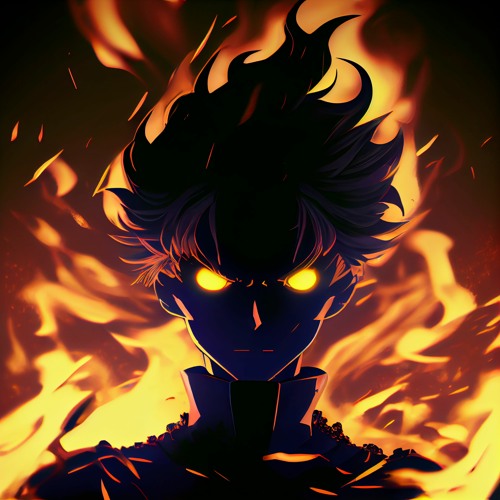The image depicts a computer-generated, cartoonish character with a distinctly anime or manga style. The figure, resembling a boy, has glowing, solid yellow eyes that radiate an intense, angry expression. His face is shrouded in shadows, making his facial details like his long, pointy nose and straight-line mouth subtly visible. He wears a high-collared jacket, which conceals part of his chin and neck, and features straps along the sides. His spiky, wild hair merges seamlessly with the vibrant flames behind him, which are a mix of orange and reddish tones, complementing the color of his eyes. The flames seem to emanate from his figure, adding a sense of dynamic energy and demented ambiance to the dark, ominous background.